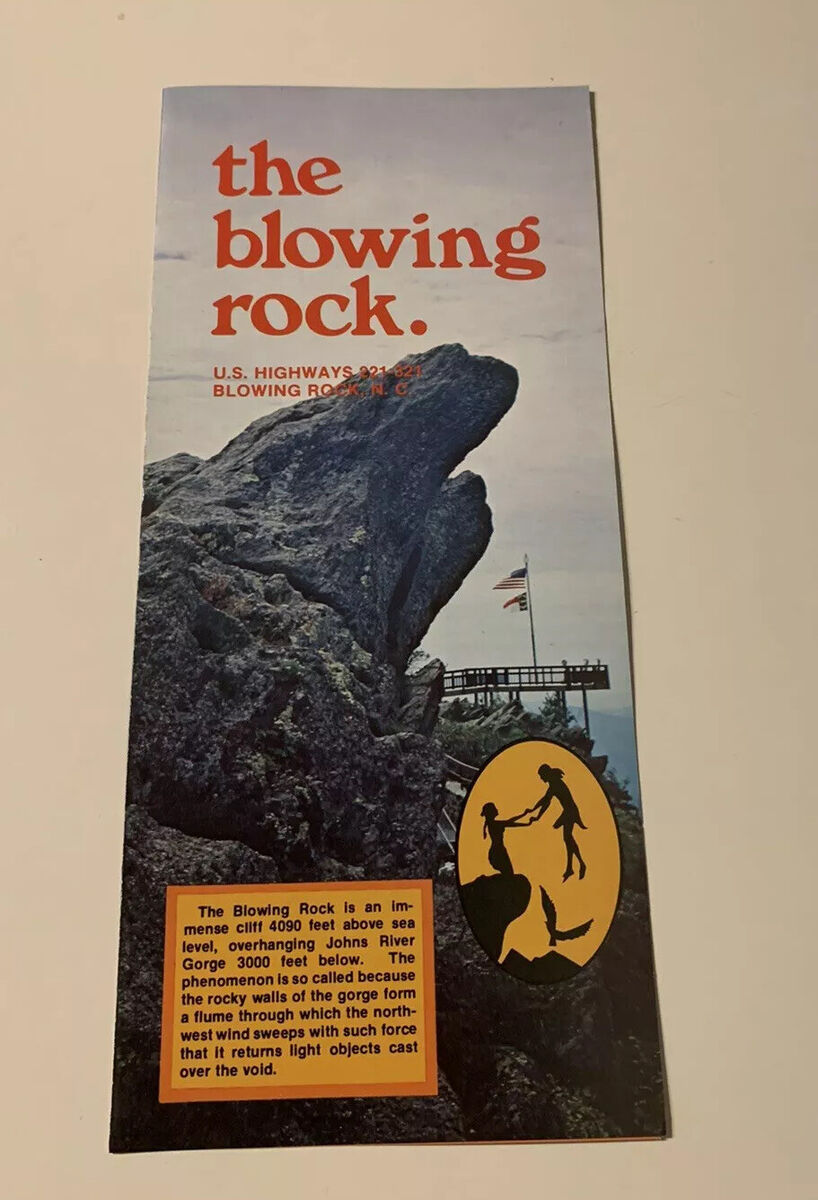The image displays a vibrant travel brochure set against a beige surface, highlighting a striking natural landmark. The brochure features a light grayish-blue background with key text in an orange font. At the top, it reads: "The Blowing Rock, U.S. Highways 221-321, Blowing Rock, North Carolina.” A prominent rocky formation extends towards the right side of the cover, accompanied by a tall flagpole sporting an American flag.

Behind the rock, you can make out a walkway dotted with numerous people. At the bottom right corner of the brochure, there is an orange oval featuring a silhouetted drawing of a woman standing on the rock, holding the hands of another person seemingly floating in midair, with an eagle soaring beneath them.

The bottom of the brochure, set against a light orange background, contains descriptive text about the landmark: "The Blowing Rock is an immense cliff 4,000 feet above sea level overhanging Johns River Gorge. The phenomenon is so called because the rocky walls of the gorge form a flume through which the northwest wind sweeps with such force that it returns light objects cast over the void." This information is critical for understanding the unique natural wonder being presented.